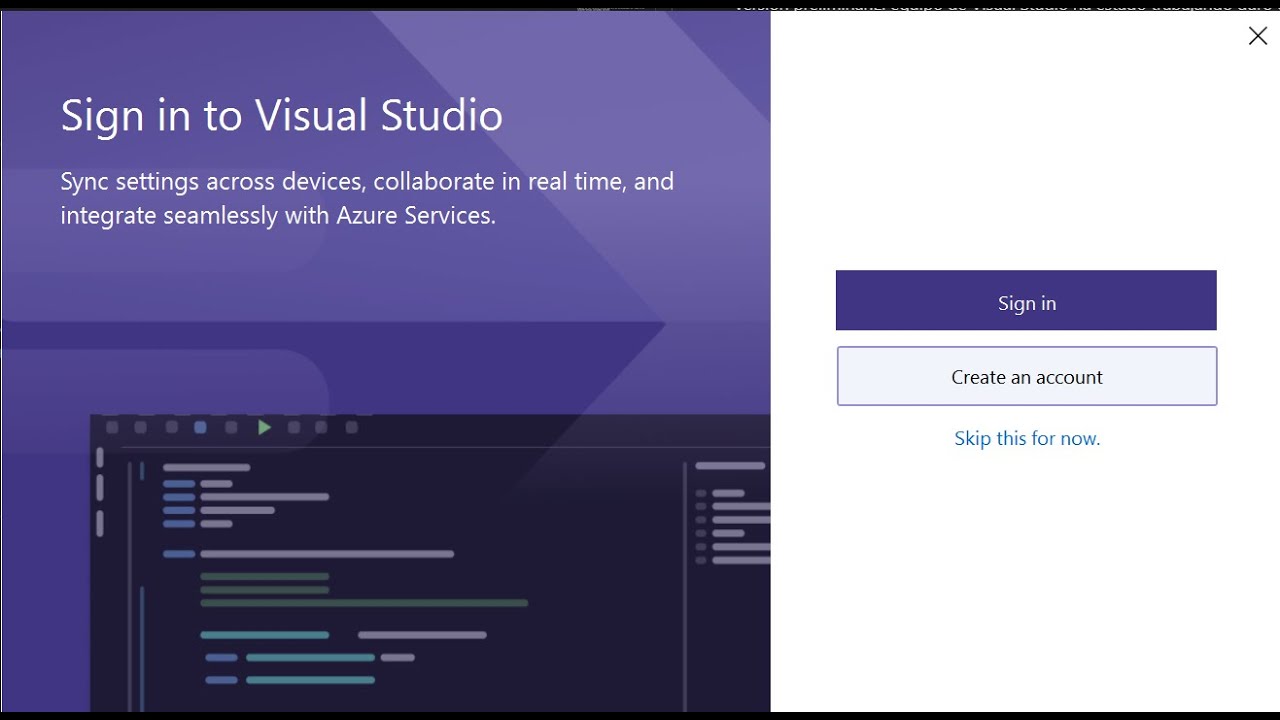The image features a sign-in screen for Visual Studio, displaying a prompt to "Sign in to Visual Studio." The screen elaborates on the benefits of signing in, including the ability to sync settings across devices, collaborate in real-time, and integrate seamlessly with Azure services. The layout is divided into two primary sections: a purple square situated above a black square, both visually representing elements of the Visual Studio interface.

To the right, there is a vertical panel with options to "Sign in" or "Create an account," accompanied by a prompt to "Skip this for now." These options are presented as two distinct buttons on a clean white background with no additional elements behind them. In the upper left corner of the screen is a small 'X,' implying an option to close the window. The overall design of the screen is rectangular.